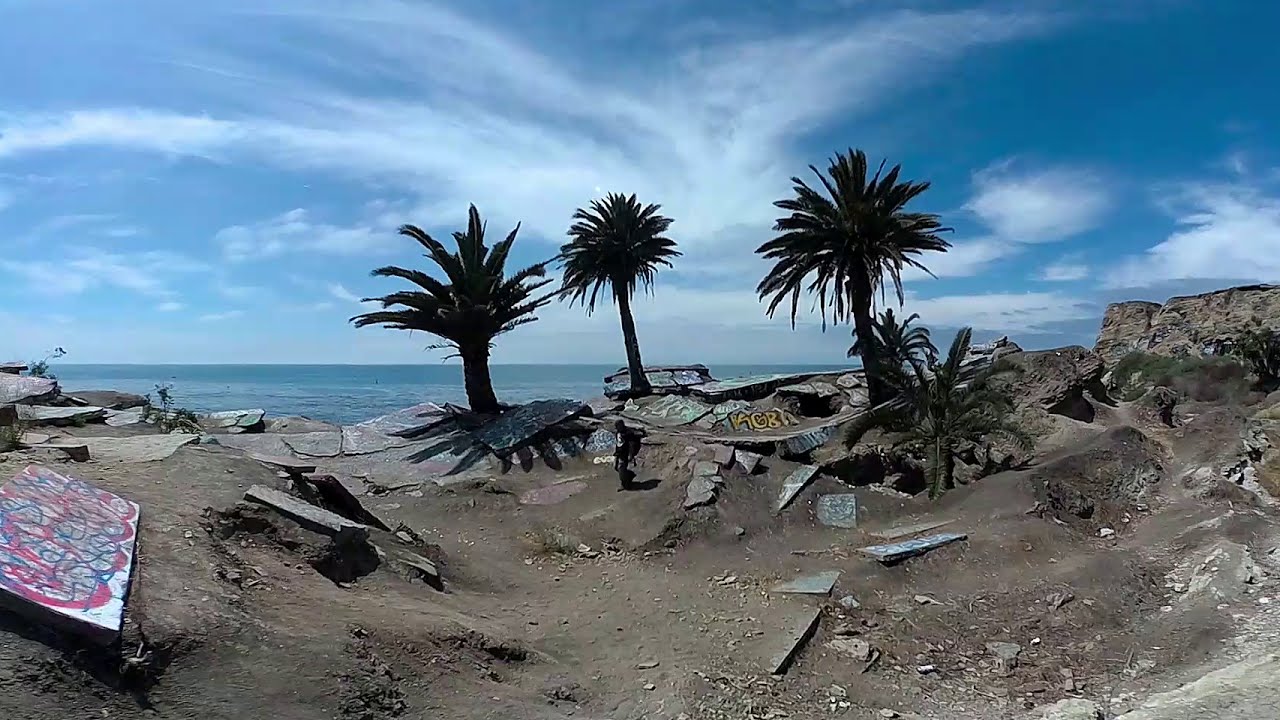The photograph depicts an abandoned beach scene dominated by dirt and rocks instead of sand. Strewn across the dirt are broken pieces of cement in varying sizes, many of which are covered in colorful graffiti, including prominent yellow text reading "KGR" on one of the larger pieces. In the center of the image, a person is walking, adding a sense of scale and solitude to the setting. The horizon showcases a vast expanse of ocean under a partly cloudy, light blue sky. The landscape is punctuated by three tall palm trees, silhouetted by shadows, and a smaller palm tree, all clustered near the center. To the left, a painted and graffitied piece of wood adds another layer of urban decay. The overall mood is one of desolation and contrast, with the natural elements of the sea and sky juxtaposed against the man-made debris and graffiti.